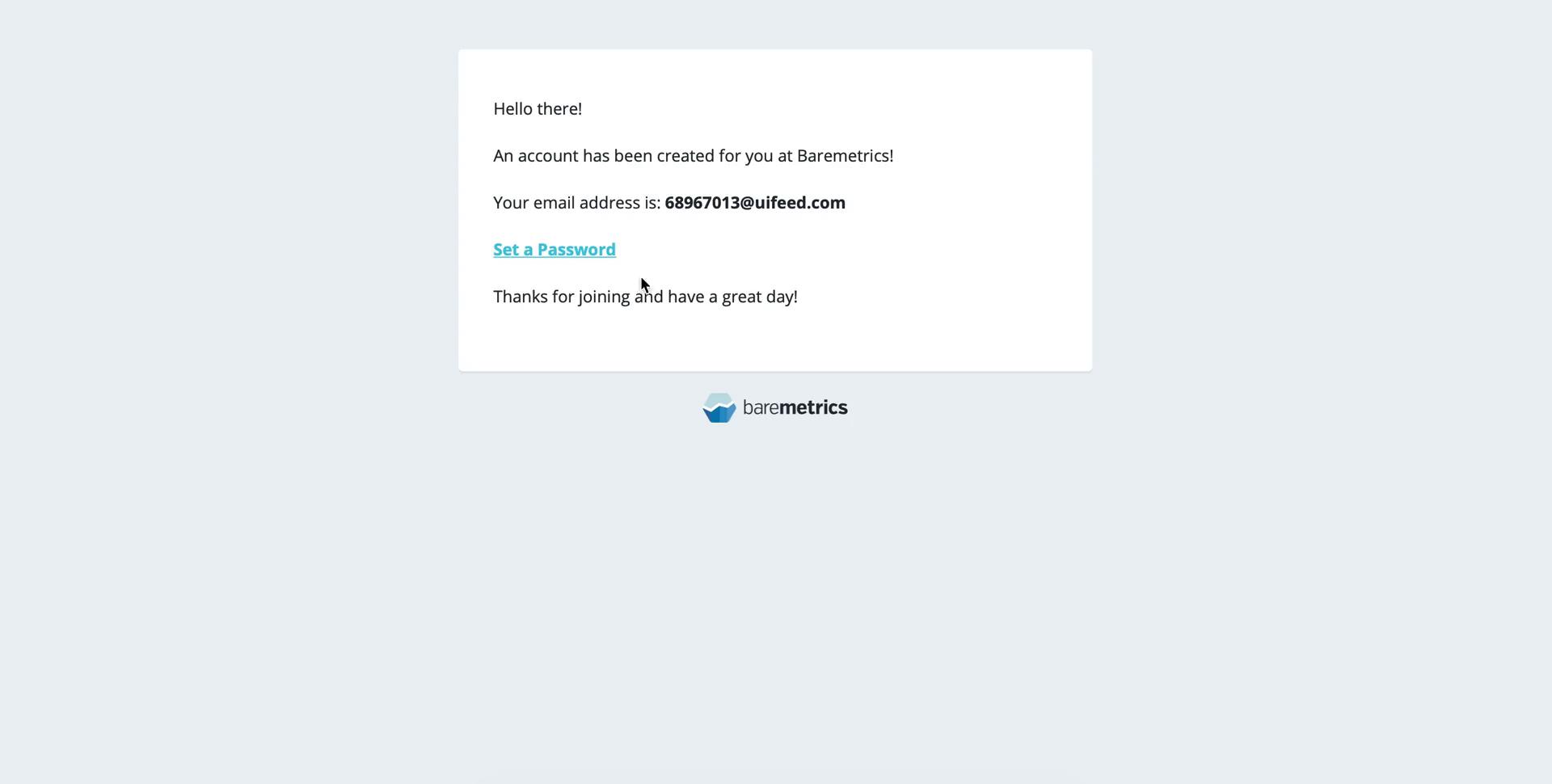The image displays a confirmation screen from the company Baremetrics. The design is clean and straightforward, featuring a single bluish light gray background without any gradients. The layout is wider than it is tall.

Positioned towards the top center is a white rectangular box. Within this box, black text reads:

"Hello there!"
"An account has been created for you at Baremetrics (spelled out as B-A-R-E-M-E-T-R-I-C-S)!"

Following this, it displays:
"Your email address is: 68967013@uifeed.com" in bold. 

Below this, there is a teal, underlined text saying "Set a password," which presumably acts as a link. 

Concluding the message in black text:
"Thanks for joining and have a great day!"

Below the white box, the company name "Baremetrics" is displayed, with "Metrics" prominently bolded. To the left of the company name is a distinct six-sided logo, divided diagonally into a light teal and a darker blue segment.

Overall, this screen confirms the creation of an account linked to a specified email address and prompts the user to set a password.